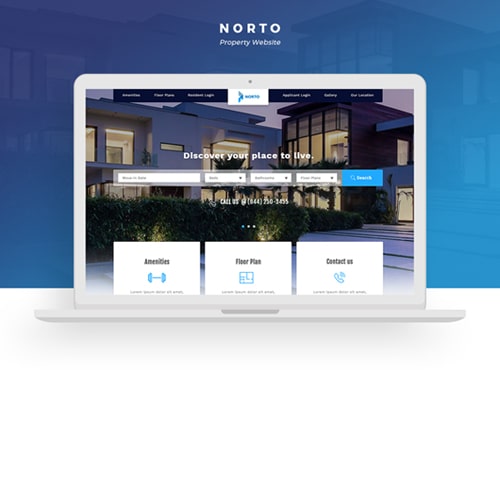The image features a bluish background with a modern housing theme. At the top center, the text "Norto Property Website" is displayed prominently. Below this, a generic laptop, resembling a MacBook, is shown with the website's homepage on its screen. The homepage showcases an image of modern houses—a white house on the left and a black house on the right, or possibly a single house with different color schemes.

In large white text, the homepage reads "Discover Your Place to Live." Below this heading, there is a search area with a blue button labeled "Search" in white text. Although partially obscured, additional options listed include "Amenities" and "Contact Us," both on white backgrounds.